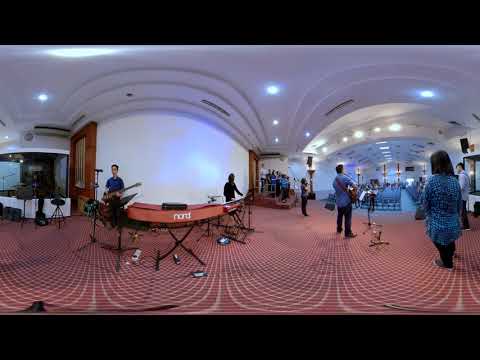The panoramic image captures a performance taking place in a church setting, viewed from the stage's perspective. The stage is adorned with red, semi-circle patterned carpeting, and has striking white vaulted ceilings with lights embedded. A church band is performing, consisting of a guitarist in a blue shirt on the left, and a keyboardist on the far left, with a notable red keyboard. To the right, there's another guitarist, and a woman in a long blue dress. In the background and off to the right, a choir—mostly dressed in blue—can be seen standing, possibly singing. This ensemble faces out over what appears to be pews arranged for a congregation. Despite the distorted perspective of the panoramic shot, the sense of a live musical performance in a church setting is clearly conveyed. The stage setup, consistent choice of blue attire, and minimal audience present suggest either a rehearsal or a smaller gathering within the church.